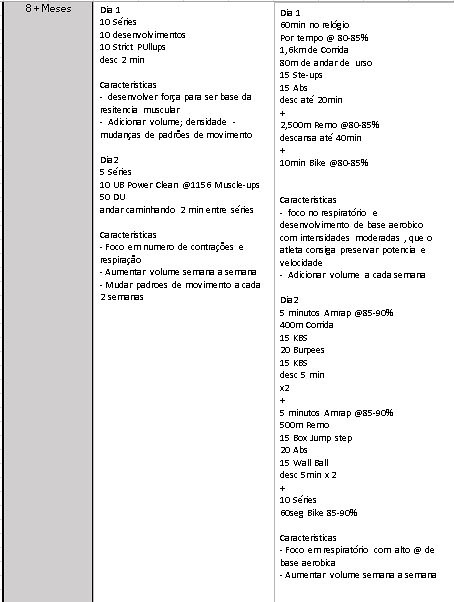The image is a black and white exercise plan not in English, potentially Spanish, displaying a list format with instructions spread across multiple columns. The first column, shaded in gray, appears to list months, indicated by "8 plus meses." The second column mentions "día 1" (day 1) and "día 2" (day 2) with various items under each day. The third column also outlines "día 1" and "día 2" with more detailed items. Notable entries include "10 minute bike" and "burpees," suggesting it's a workout regimen. Despite its blurriness, the document provides a structured schedule for different days, implying a sequential fitness plan or routine.